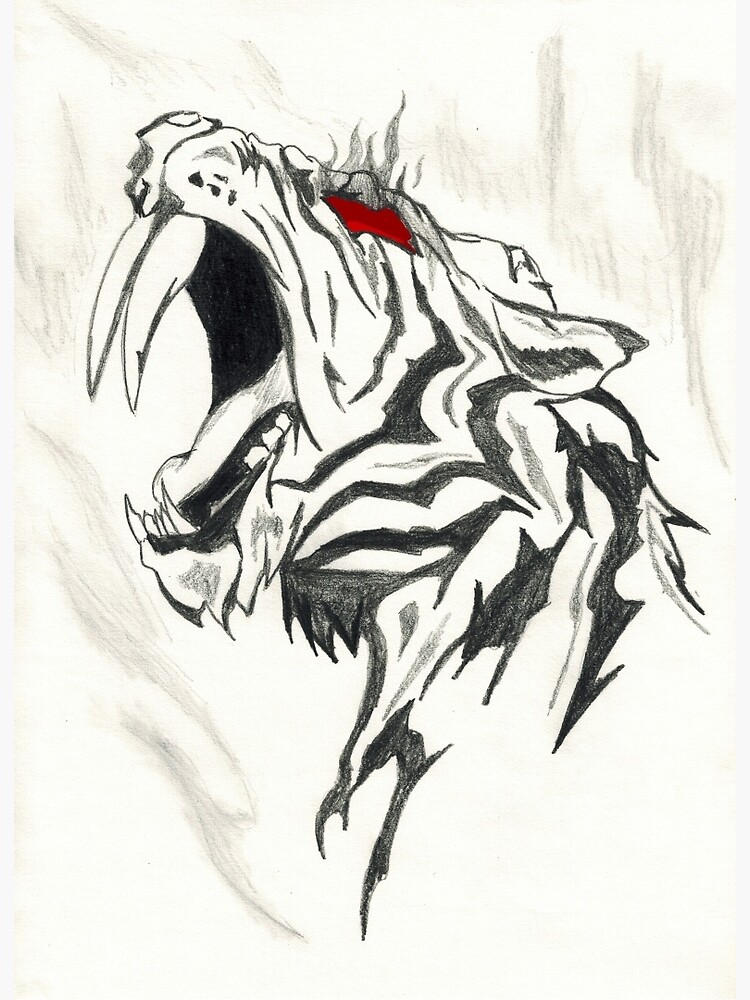This is a detailed black and white pencil drawing of a roaring saber-toothed tiger, facing left. The piece is rendered on an off-white sheet of paper, with intricate pencil shading to bring out the textures and shadows. The tiger's mouth is wide open, displaying two long, prominent fangs at the top and sharp teeth along the bottom. The inside of its mouth is shaded black, revealing its tongue. The tiger's powerful neck and tense shoulders add to the impression of a fierce roar. Remarkably, its eye is colored a striking red, adding a splash of color to the monochromatic scene. The detailed striping on the tiger extends from its head down to the top of its neck, with visible pencil textures enhancing its lifelike appearance. The background features a subtle blend of white and gray shading that frames the tiger, emphasizing its dramatic presence.